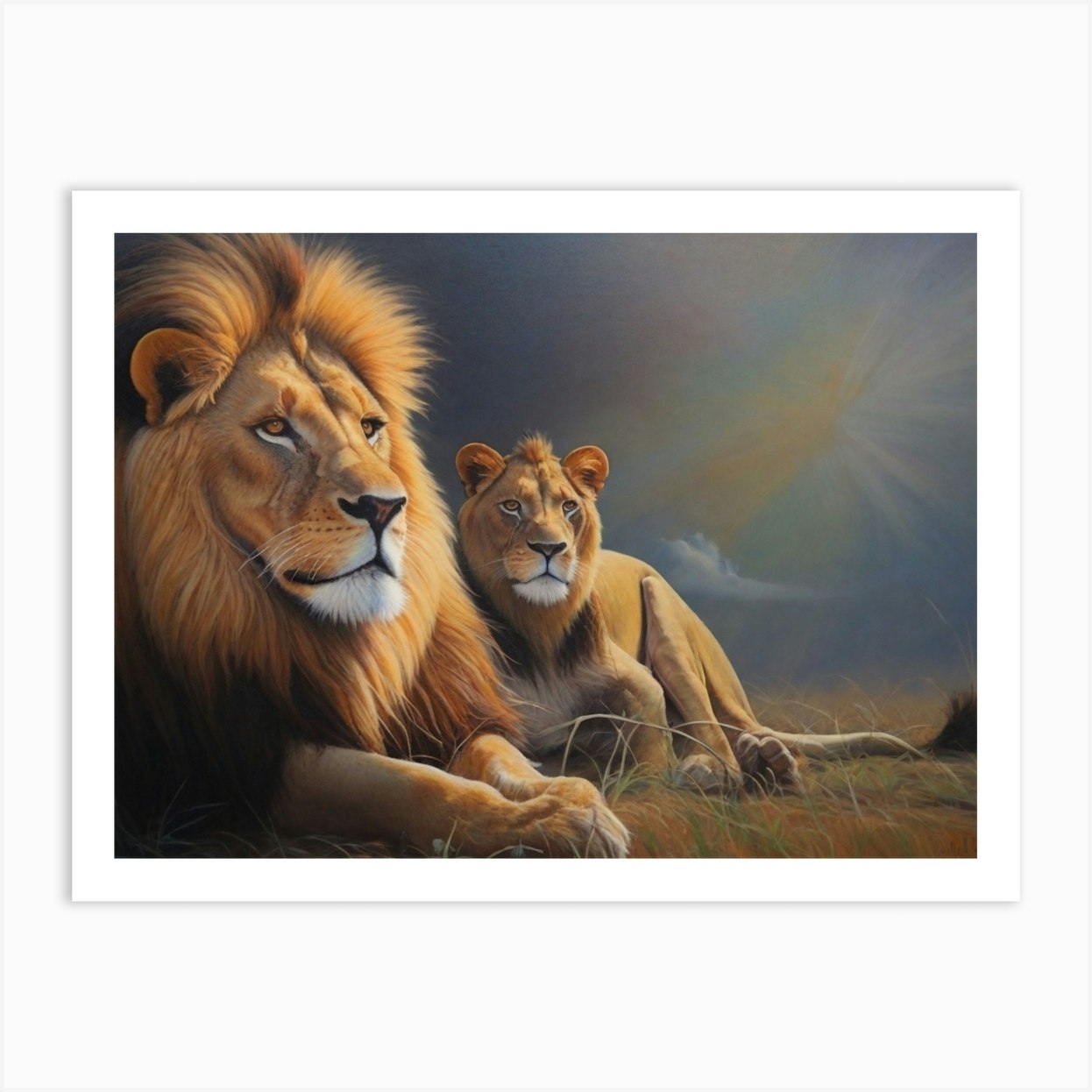The digital artwork depicts a stoic male lion and a serious female lioness lying down in a sparsely grassy area. The male lion, identifiable by its prominent mane, is positioned on the left, while the lioness, with her mane-less profile, is on the right. Both lions have serious expressions, indicating they might be in a hunting or alert mood. The background features a white sky with a semi-large puffy cloud and a sunburst above and to the right of the cloud, casting a golden light that illuminates the scene. The setting is minimalistic, with only a few patches of green and brown grass, and no visible text. The painting is displayed against a white wall, adding to its simple yet majestic presentation.